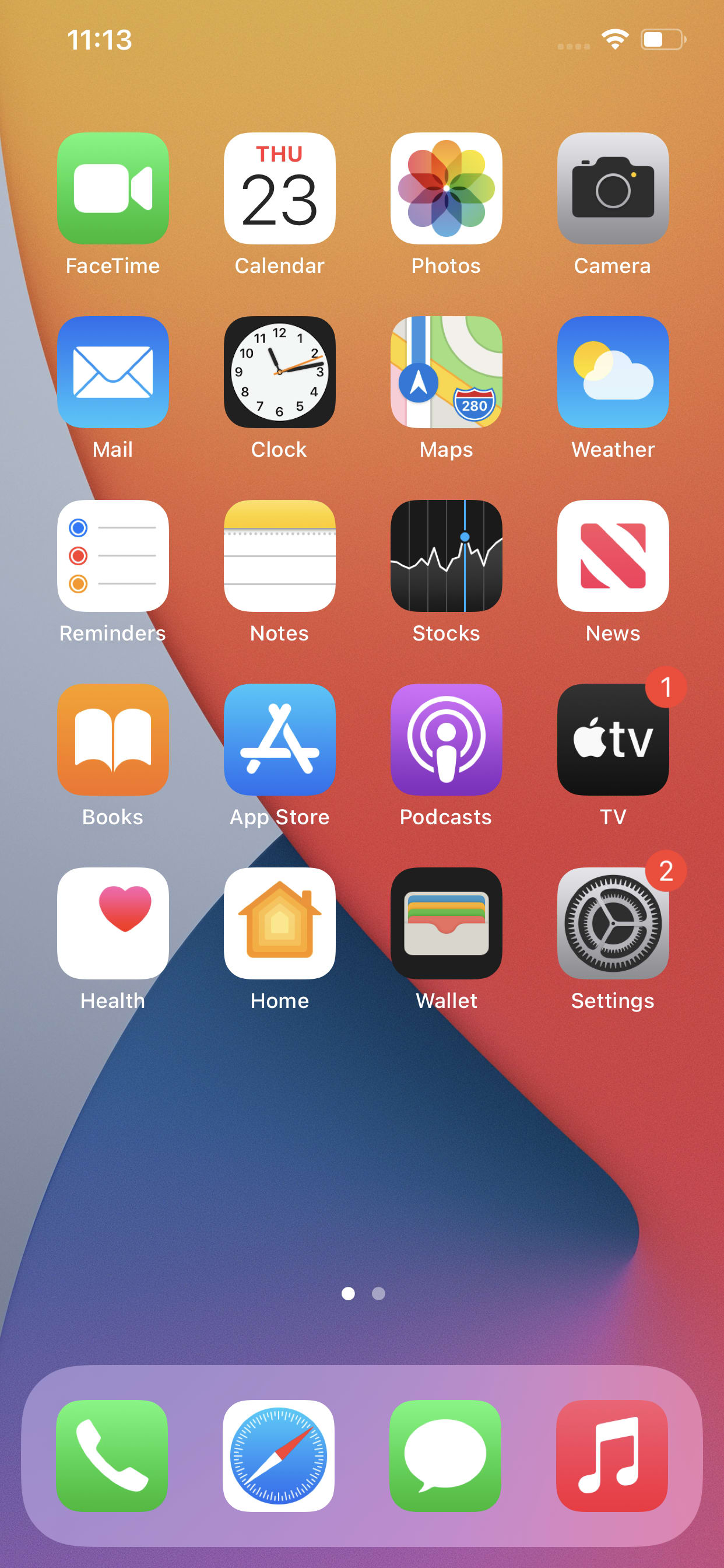This image depicts the home screen of a smartphone, meticulously showcasing various elements and icons. In the top left corner, the time is displayed as 11:13. On the right side, there are indicators for battery level, WiFi signal strength, and cellular service bars, providing essential status information at a glance.

The background image is a captivating blend of colors, including shades of orange, blue, lighter blue, and a touch of purple at the bottom, creating a visually appealing backdrop.

A diverse array of app icons is organized on the screen. Starting from the top, there is a green FaceTime icon featuring a camera symbol. Adjacent to it is a calendar icon showing "Thu" for Thursday and the number 23. Other notable icons include the Photos app, Camera, Mail, Clock, Maps, and a blue Weather icon depicting a sun and cloud.

Additional apps displayed are Reminders, Notes, Stocks, News, Books, App Store, Podcasts, TV, Health, Home, Wallet, and Settings. 

At the very bottom of the screen, a dock contains four frequently used icons: a green Phone icon, a blue Safari browser icon, a green Messages icon, and a pink Music icon. This arrangement ensures quick access to these essential applications.